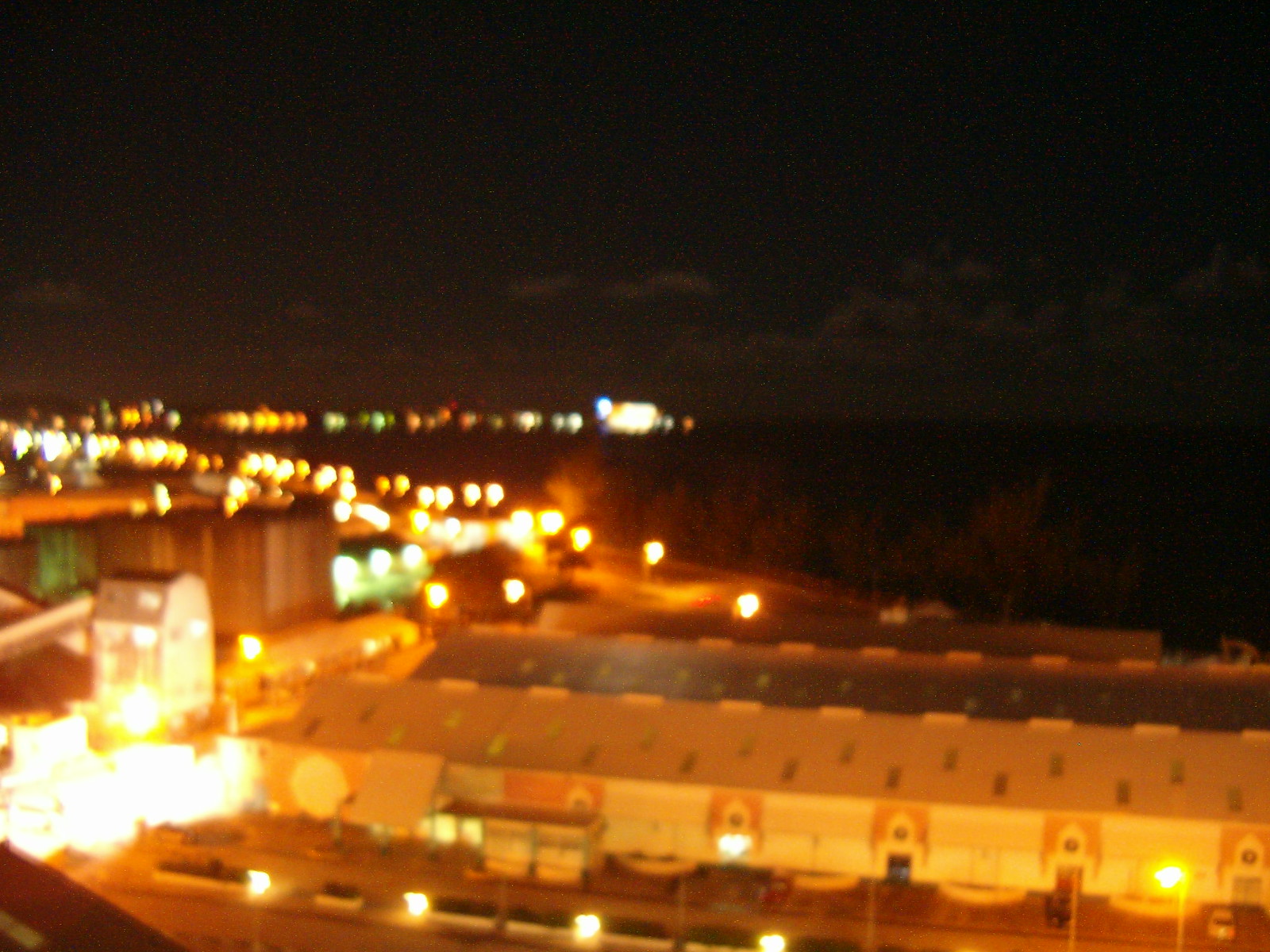This photo appears to be an overhead, slightly blurry image likely taken from a bridge, showcasing a residential area with city lights in the background. The focus is on several white condo or townhouse-style housing units, distinguished by brown framing around the doors which also feature a distinctive round design at the top. The roofs of these structures are brown with multiple skylights cut into them. The background reveals a cluster of city and traffic lights in hues of yellow, green, red, and white, extending from the left side of the photograph towards the center. The upper part of the image captures a dark night sky. Towards the bottom right, there is a two- to three-story housing structure with a barn-style roof, illuminated by a brightly lit area in the lower right corner.